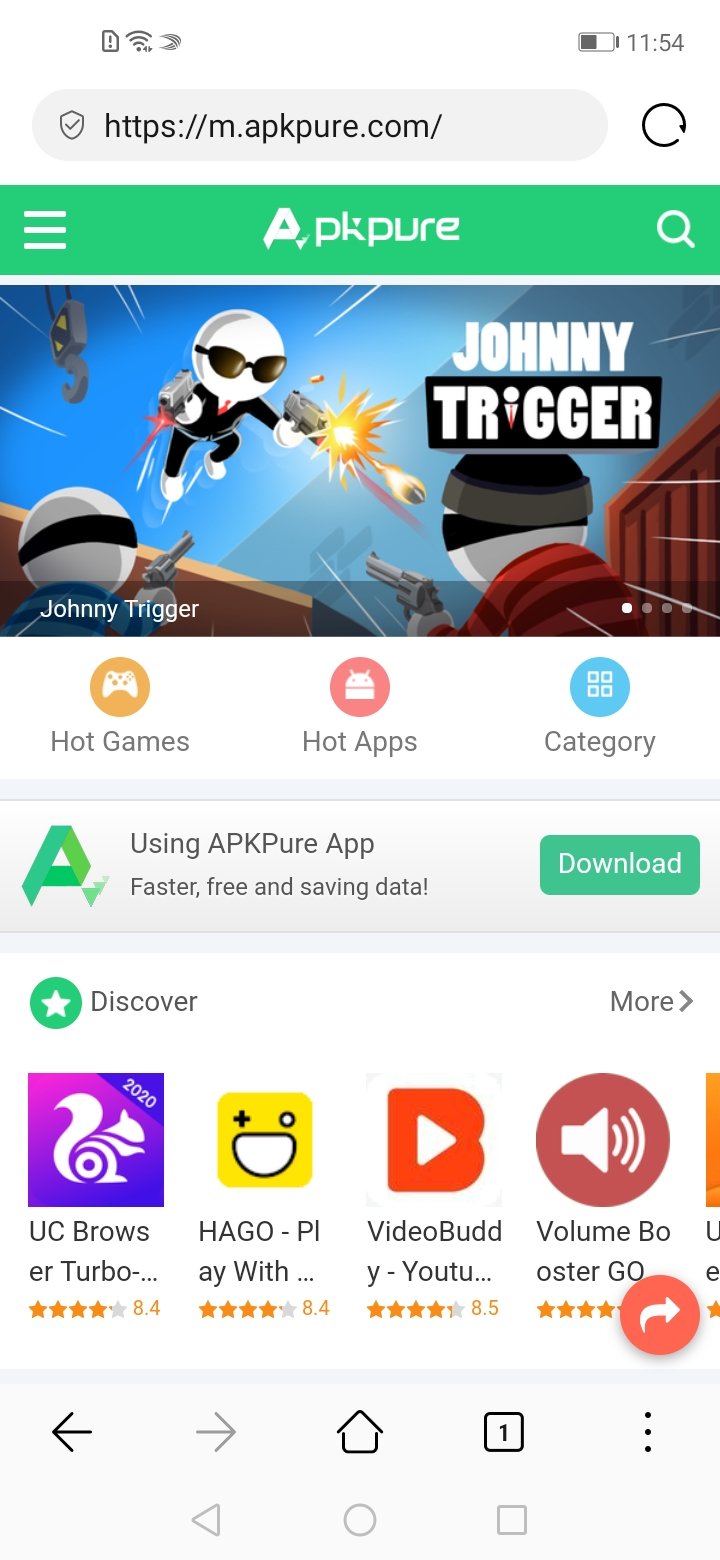The image displayed on the cell phone screen shows a detailed view of a mobile webpage. In the top-right corner, the status bar shows the time as 11:54 along with the Wi-Fi signal icon and battery level. To the left of these symbols, there are additional icons indicating other notifications.

The web browser is open to the URL "https://m.apkpure.com/", indicated in a grey-shaded address bar which also includes a small half-circle on the right side. The website header is a green section featuring a white magnifying glass icon and the word "Acpeer" written in white.

The main content area features a theme for the game "Johnny Trigger." The game illustrates a white space character wearing glasses, a black suit, and a red tie, depicted mid-air while shooting at two individuals who appear to be robbers, identified by the black bands around their eyes and their striped outfits—one in red stripes and the other in blue.

Below this game section, there are categories labeled "Hot Games," "Hot Apps," and "Category," each accompanied by their individual circular icons. The APKPure app offers a download option emphasizing "faster, free, and saving data," along with a "Discover" section, marked by a green circle with a white star inside.

Among the apps showcased for discovery are:
1. "UC Browser Turbo" with an animated squirrel logo.
2. "HeigopieAwe," represented by a yellow square emoji with one eye as a plus sign, another as a white circle, and a large white mouth.
3. An app featuring a big "B" with a white triangle in the center.
4. "Volume Booster GO," symbolized by a speaker emitting signal waves.
5. "Video Bud YouTube," all of which have ratings ranging from 8.4 to 8.5, displayed next to an orange circle with a white arrow.

At the bottom of the page, there are navigation arrows on the left and right sides, with the left arrow highlighted. Additionally, a house icon, a square with the number one, and a menu icon with three dots are visible on the left side of the screen.